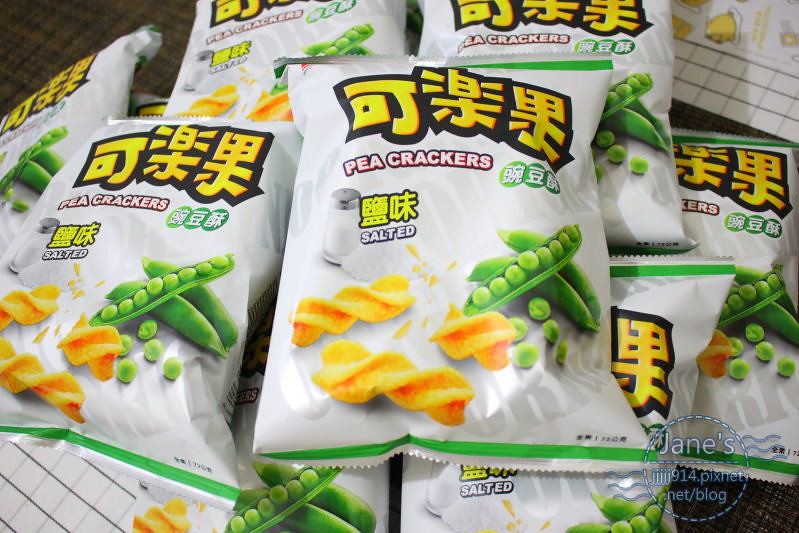The photograph features multiple bags of a snack product displayed on a wooden table. Each white bag is adorned with a green trim at the top and bottom edges and has a ruffled texture. Prominently, at the top of the bag, there are large Asian letters in a yellow color with a black outline, and below that, the English words "Pea Crackers" are displayed in a red and white font, followed by the word "Salted." An illustration on the bag depicts the twisted, tan-colored crackers accompanied by two closed pea pods, an open pea pod, individual peas scattered around, and a salt shaker positioned to the left. The contents appear identical across all bags, and they are piled up for the photograph. Additionally, there is some sort of paper beneath the bags on the right-hand side, and a watermark at the bottom reads, “Jane’s Pig’s Net Blog.” Overall, there are about eight bags arranged in the image.